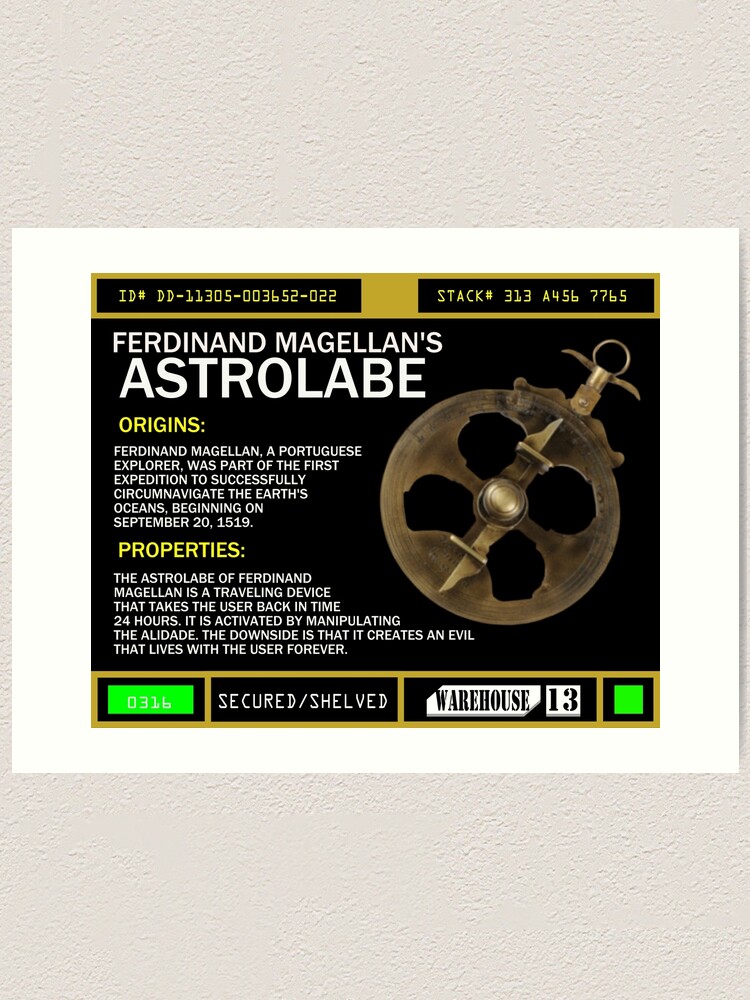The image showcases a graphic design against a textured white-painted drywall background. At the center is a white rectangle containing a black box with a variety of text elements. At the top of the box, in gold lettering, is the ID number "DD-11305-003652-022." Adjacent to this is the stack number "313A4567765." Below, in white capital letters, the text reads "Ferdinand Magellan's Astrolabe." Continuing in smaller yellow and white text, the caption details:

"Origins: Ferdinand Magellan, a Portuguese explorer, was part of the first expedition to successfully circumnavigate the Earth's oceans, beginning on September 20th, 1519.

Properties: The astrolabe of Ferdinand Magellan is a traveling device that takes the user back in time 24 hours. It is activated by manipulating the Alidade. The downside is that it creates an evil that lives within the user forever."

To the right of this descriptive text is an image of the device itself, a brass circular astrolabe featuring several intricate components. The astrolabe has a key ring-like attachment at the top and multiple nested circles with protruding points. Below this detailed description, a section in green font reads "0316" and "secured/shelved," with "Warehouse 13" written in black text on a white background, followed by a green square. This composition effectively blends historical context with the fictional properties attributed to the astrolabe, tying it into the "Warehouse 13" series.